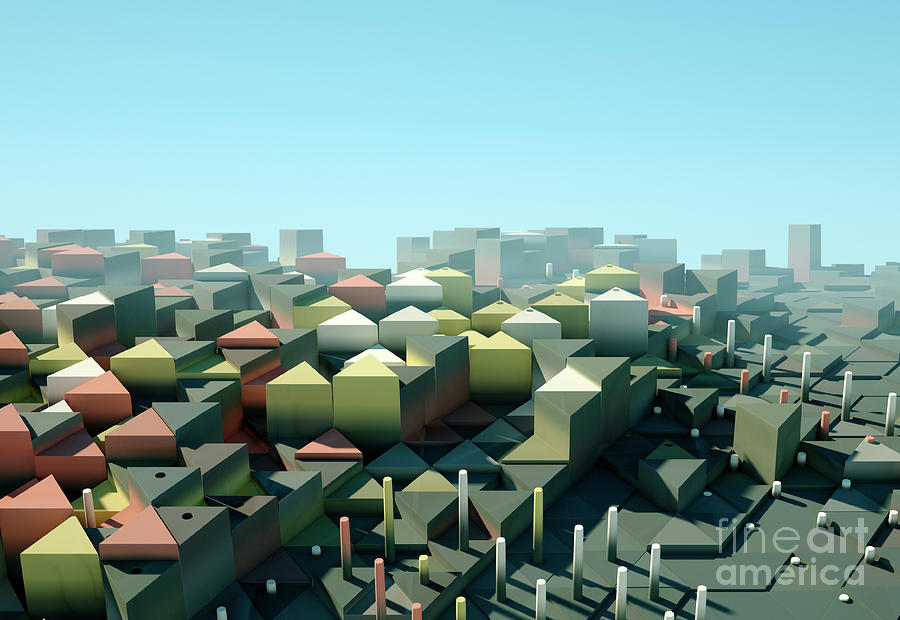This detailed 3D-rendered and computer-generated image showcases an abstract cityscape formed by colorful geometric shapes reminiscent of wooden blocks on pegs. The illustration is divided into two distinct sections: the upper half features a gradient blue sky that becomes lighter towards the bottom, and the lower half is populated with a series of triangular and square shapes, creating a visually striking juxtaposition. The triangular forms, concentrated in the front left, mimic pyramids in rusty red-orange, white, charcoal black, light yellow, and occasionally green and pink. They transition into square-shaped building-like structures towards the background, implying a layered cityscape of various heights and dimensions. Smaller pole-shaped objects in the same color palette (yellow, white, and pink) are scattered around the front and right areas. The entire scene, with its vibrant colors and wooden toy-like appearance, is designed to evoke a playful yet sophisticated abstract interpretation of a city. The text "Fine Art America" is subtly placed in the lower right corner of the image.